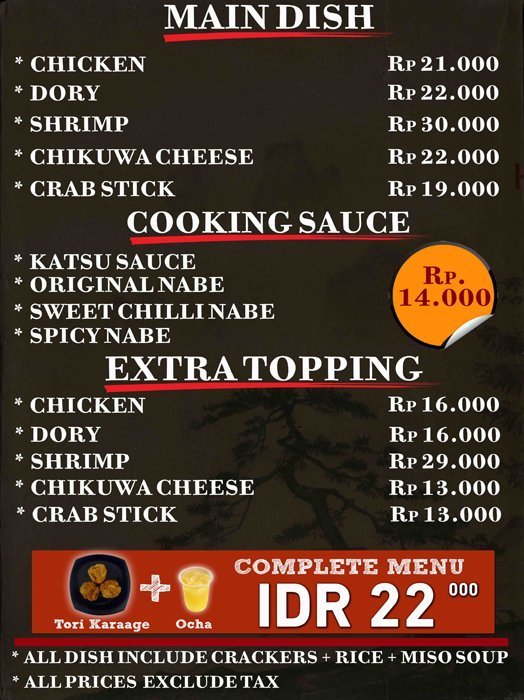The menu, presented in a portrait orientation with a black background and white text, is divided into three sections:

1. **Main Dish**: 
   - The section title "MAIN DISH" is in uppercase, white letters, underlined in red.
   - Listed items include:
     - Chicken: Rp21.000
     - Dory: Rp22.000
     - Shrimp: Rp30.000
     - Chikuwa Cheese: Rp22.000
     - Crab Stick: Rp19.000

2. **Cooking Sauce**:
   - The section title "COOKING SAUCE" is also in uppercase, white letters, underlined in red.
   - Listed sauces include:
     - Katsu Sauce
     - Original Nabe
     - Sweet Chili Nabe
     - Spicy Nabe
   - To the right, there is a gold circle with "Rp14.000" printed in red.

3. **Extra Topping**:
   - The section title "EXTRA TOPPING" is in uppercase, white letters, underlined in red.
   - Listed items include:
     - Chicken: Rp16.000
     - Dory: Rp16.000
     - Shrimp: Rp29.000
     - Chikuwa Cheese: Rp13.000
     - Crab Stick: Rp13.000

A red horizontal strip at the bottom includes a photograph of a beer and the text:
   - "COMPLETE MENU" in bold white letters, priced at IDR22,000.
   - Below, in white text: "All dish include crackers, rice, miso soup."
   - Finally: "All prices exclude tax."

The combination of graphic design typography and photography makes this menu visually appealing and informative.